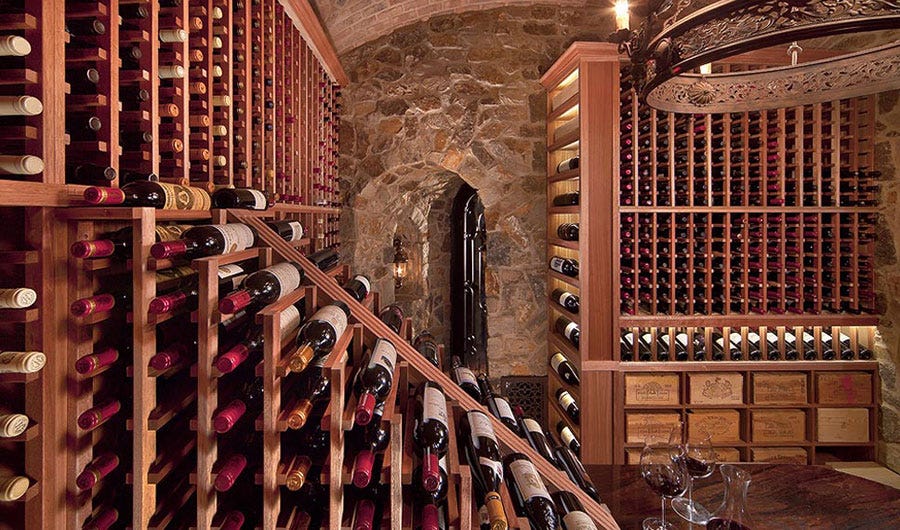This image captures a beautifully rustic wine cellar with robust stone walls. The cellar features an extensive collection of wine bottles meticulously stored in elegant, wooden wine racks that line the room. The racks not only serve as storage but add a warm, wooden charm to the space. At the bottom of one of these racks, there are practical drawers, adding an element of functionality. 

Prominently, a large wine rack graces the left wall while another substantial rack is positioned on the right side. In the center, a wooden table holds two wine glasses and a wine decanter, which appears to contain a small amount of red wine, hinting at a recent or forthcoming tasting session. 

An arched doorway adds architectural interest to the scene, while a lantern-style lamp affixed to the stone wall provides ambient lighting. Overhead, a round chandelier dangles from the ceiling, casting a warm glow over the room and enhancing its cozy, inviting atmosphere.